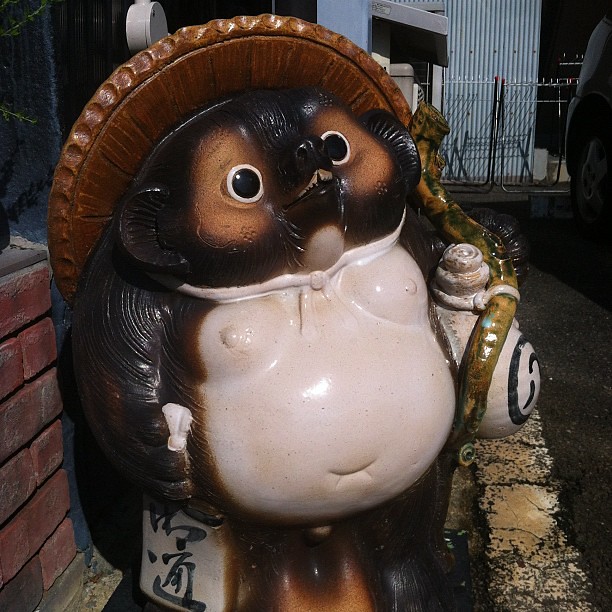In this image, we observe an outdoor scene set on an asphalt road, flanked by a brick wall on the left and a gate with barbed wire in the background, possibly adjoining a commercial building. Central to the image is a detailed statue of an anthropomorphic creature, appearing rodent-like, perhaps a mix of a squirrel, bear, and beaver. The statue showcases intricate features: it stands upright, has a large white belly with a visible belly button and rounded chest area, and sports a wide, brown sombrero-like hat secured by a tie. The creature has dark brown fur with lighter brown around the eyes and black eyes. Looking slightly towards us, it holds a green stick with a white canister featuring a black symbol in its right hand (our left). In its left hand (our right), it grasps a white sign adorned with Asian characters. The colors in the image include black, white, brown, tan, off-red, green, and light blue, indicating a bright, clear setting in the middle of the day.